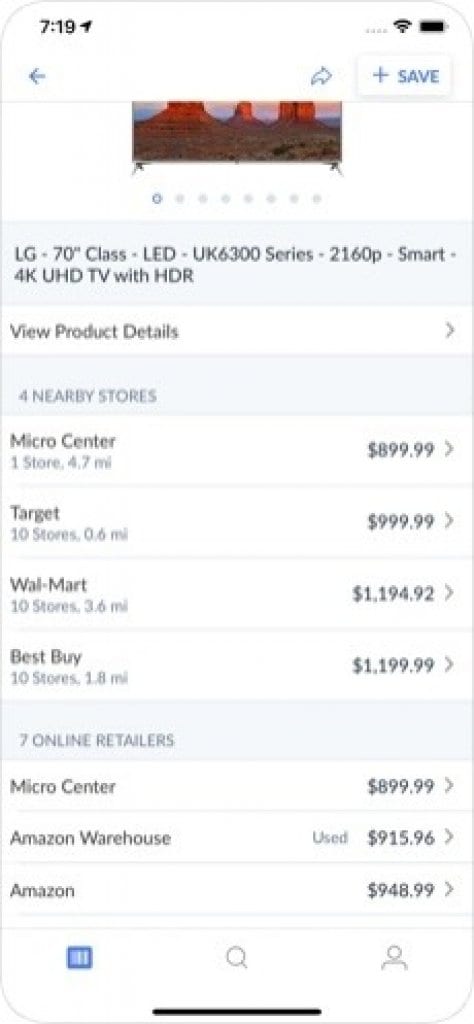The image depicts a smartphone screenshot. The top portion of the screenshot shows a partially visible photograph, likely of reddish-colored rock formations emerging from a brown sandy landscape, set against a vivid, colorful sky.

Below the image, a rectangular box displays the product information for an "LG 70-inch Class LED UK6300 Series 2160p Smart 4K UHD TV with HDR". Below this, there is a "View Product Details" link.

The screenshot details the availability and pricing of the TV at nearby stores:
1. Micro Center: 1 store, 4.7 miles away, priced at $899.99.
2. Target: 10 stores, 0.6 miles away, priced at $999.99.
3. Walmart: 10 stores, 3.6 miles away, priced at $1,194.92.
4. Best Buy: 10 stores, 1.8 miles away, priced at $1,199.99.

Additionally, there are listings for seven online retailers, of which three are visible:
1. Micro Center: $899.99.
2. Amazon Warehouse: $915.96 (used).
3. Amazon: $948.99.